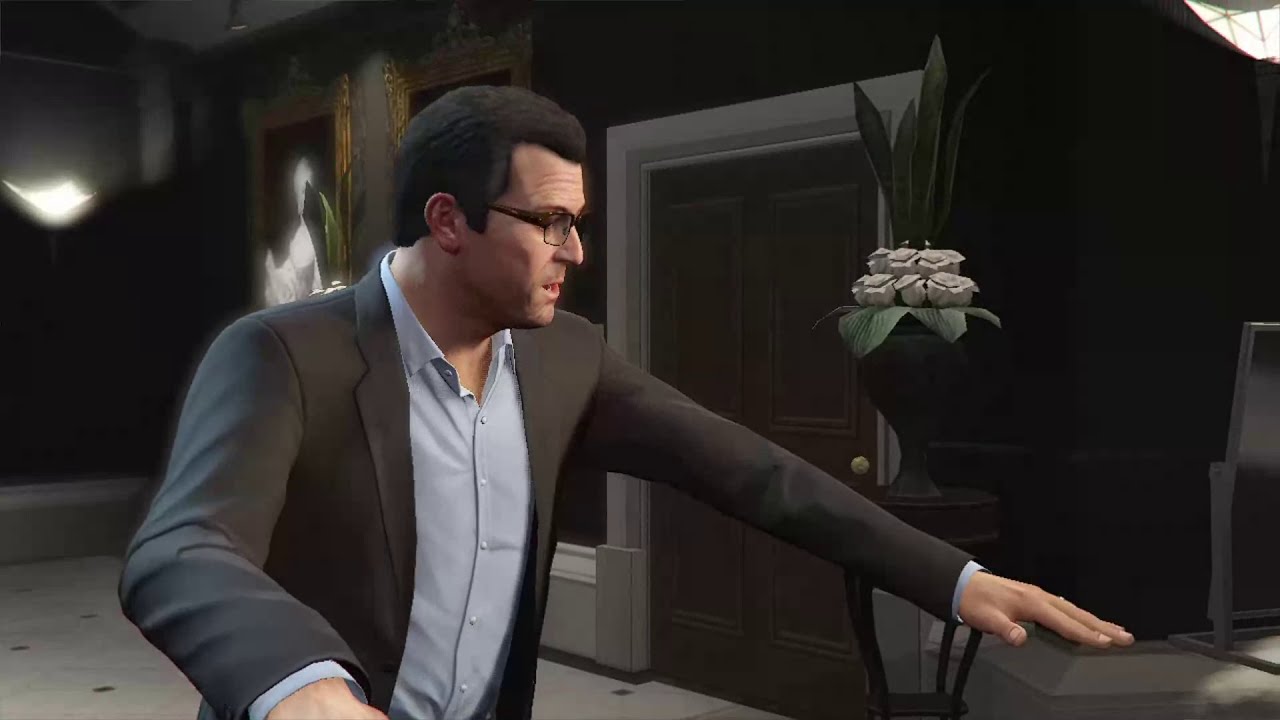In this detailed, realistic video game screenshot, a male character resembling Pierce Brosnan stands in what appears to be a dimly lit mansion hallway. The man wears a gray suit jacket over a light blue collared shirt with the top button open. He has short dark hair and thick-framed glasses. His left arm is outstretched, possibly resting on a piece of furniture.

The setting includes a dark brown door with a gold doorknob, framed by white molding, located to the left of the character. To the right of this door stands a dark wooden pedestal table adorned with a black vase containing a lush floral and leaf arrangement. Behind the character, viewers can see a tiled floor, baseboards, and a wall sconce that casts a soft glow. The walls are decorated with framed paintings, adding to the ambiance of the scene.